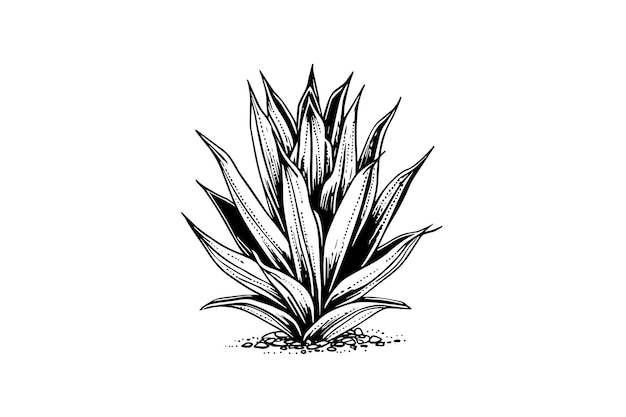This black and white graphic depicts a plant with thin, narrow, spiky leaves that radiate from a central point. The plant is rooted in a ground composed of small rocks and pebbles, suggesting a rugged environment. The leaves, notable for their sharp tips, extend both sideways and upwards, resembling the structure of a snake plant or mother-in-law's tongue. The surface of the leaves features small dotted lines, adding texture to the image. The plant appears bushy with no flowers, consisting entirely of elongated, pointed leaves that vary in shading, perhaps to indicate light and shadow. Overall, it appears to be a low-growing plant, only a few inches taller than it is wide, with an abundance of narrow, spiky leaves.